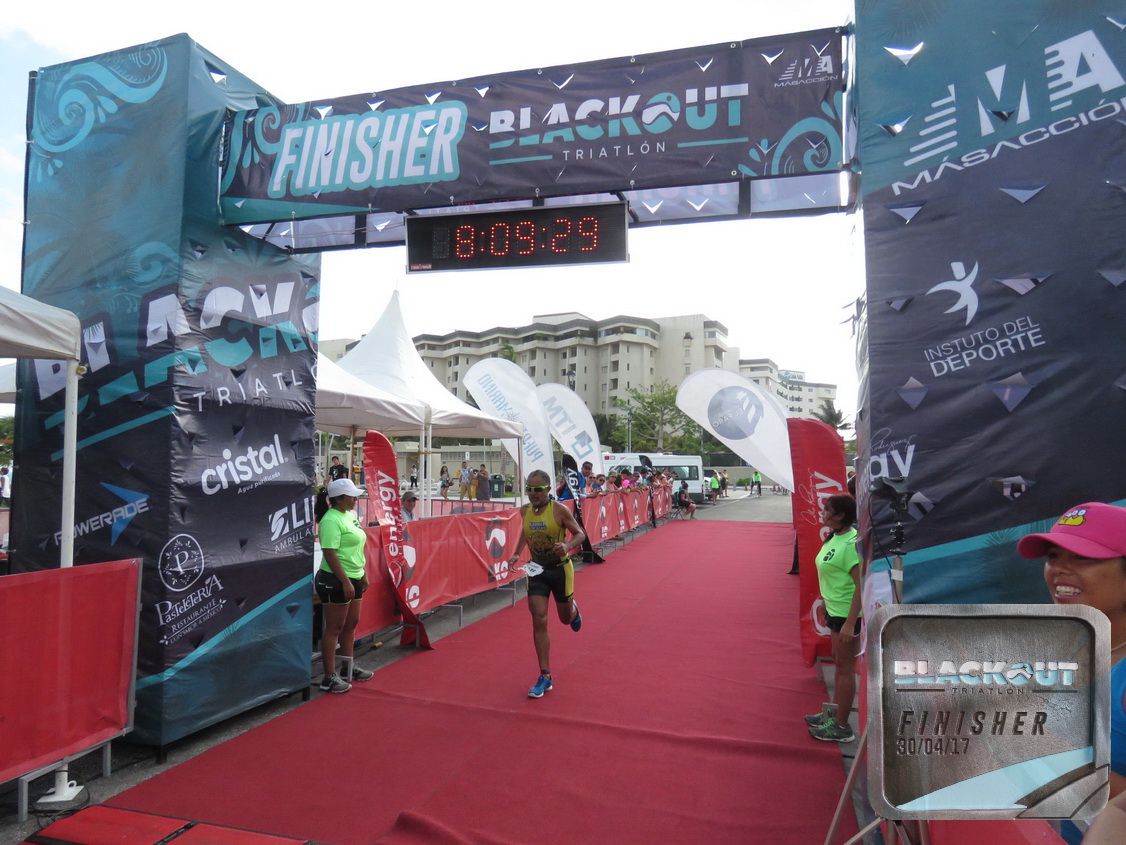The image captures the dramatic moment of a race finish line. A red carpet runs down the center, flanked by metal railings covered in red banners. Towards the end, two metal scaffoldings wrapped in banners support a crossbeam that holds a central LED timer displaying the time 8:09:29 in bright orange lights. A woman in a yellow running outfit and blue tennis shoes is crossing the finish line, observed by two women in bright green shirts standing at the base of the scaffoldings. The background reveals spectators along the race line, large structures that appear to be a hotel or resort, and multiple white tents, contributing to the vibrant finish line atmosphere. Signs reading "finisher," "blackout," and "triathlon" are visible along the sides, adding context to the event.